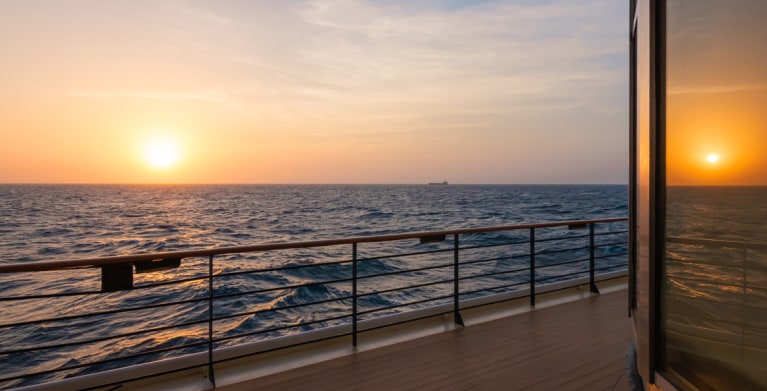The photograph, taken from the deck of a boat, presents a captivating sea view during what appears to be a sunset. The image is wide, horizontal, and rectangular, capturing the scene in intricate detail. In the foreground, the rich brown wooden deck descends slightly, leading to a dark brown metal railing. This railing, standing about 3 to 4 feet tall, is composed of horizontal bars connected by evenly spaced vertical poles. Just beyond the railing lies the vast expanse of the ocean, its blue waters adorned with waves and capturing the essence of the sea's ceaseless beauty.

Dominating the horizon, the sun is either setting or rising—its position ambiguous but striking. Encircled by a hazy halo, the sun casts a palette of orange, red, and pink hues across the sky, mirrored by the surrounding clouds. On the right edge of the image, reflective tall windows from the boat capture and duplicate the sunset's glow, creating an illusion of two suns and intensifying the scene's ethereal quality. A ship is faintly outlined on the distant horizon, adding a sense of scale and solitude to the breathtaking maritime vista.